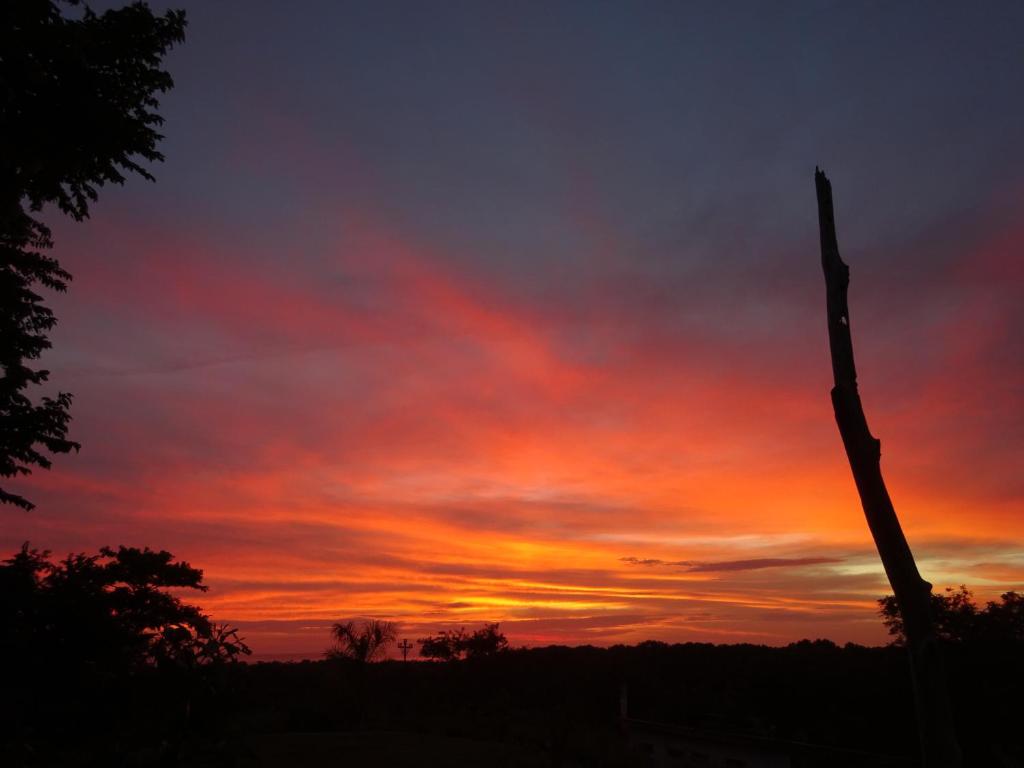The photograph captures a serene sunset over a tranquil landscape. The sky transitions beautifully from deep, muted blue at the top to vibrant purples, pinks, and finally to rich oranges and yellows near the horizon. The left side of the image is adorned with the dark silhouettes of a tall tree's leaves extending into the frame's top left corner, and below them, a shorter tree. The right side features a prominent tree stump, entering diagonally from the bottom right corner. The landscape is mostly in shadow, creating a stark contrast with the colorful sky. Small, darkened trees and bushes dot the background, their outlines just visible against the vibrant sunset, which is the main focus of this striking image.